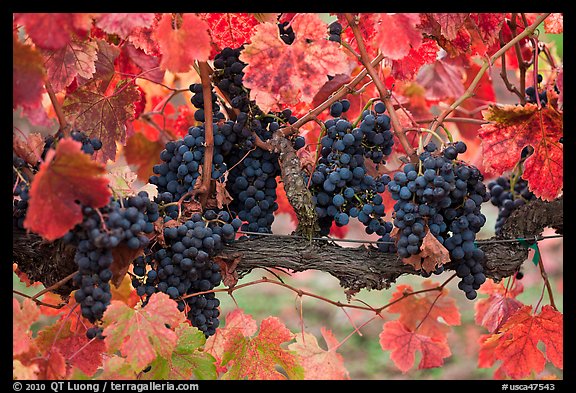This image, framed with a black border, captures a vibrant autumn scene. In the background, the leaves are transitioning to rich hues of crimson red and orange, signaling the change of seasons. A thick, brown branch runs horizontally from the left to the right side of the picture, supporting several clusters of dark purple grapes. The lush, grape-colored bunches, numbering around six to eight, hang prominently from the vine, accompanied by predominantly red leaves with a few green ones intermixed, especially in the lower left corner of the image. Small flowers are intertwined among the grapes, adding to the scene's rich texture and visual appeal. The bottom of the image features the copyright notice "2010 qtluong.com" on the lower left and the hashtag "#USCA47543" on the lower right, all encompassed within the black frame.